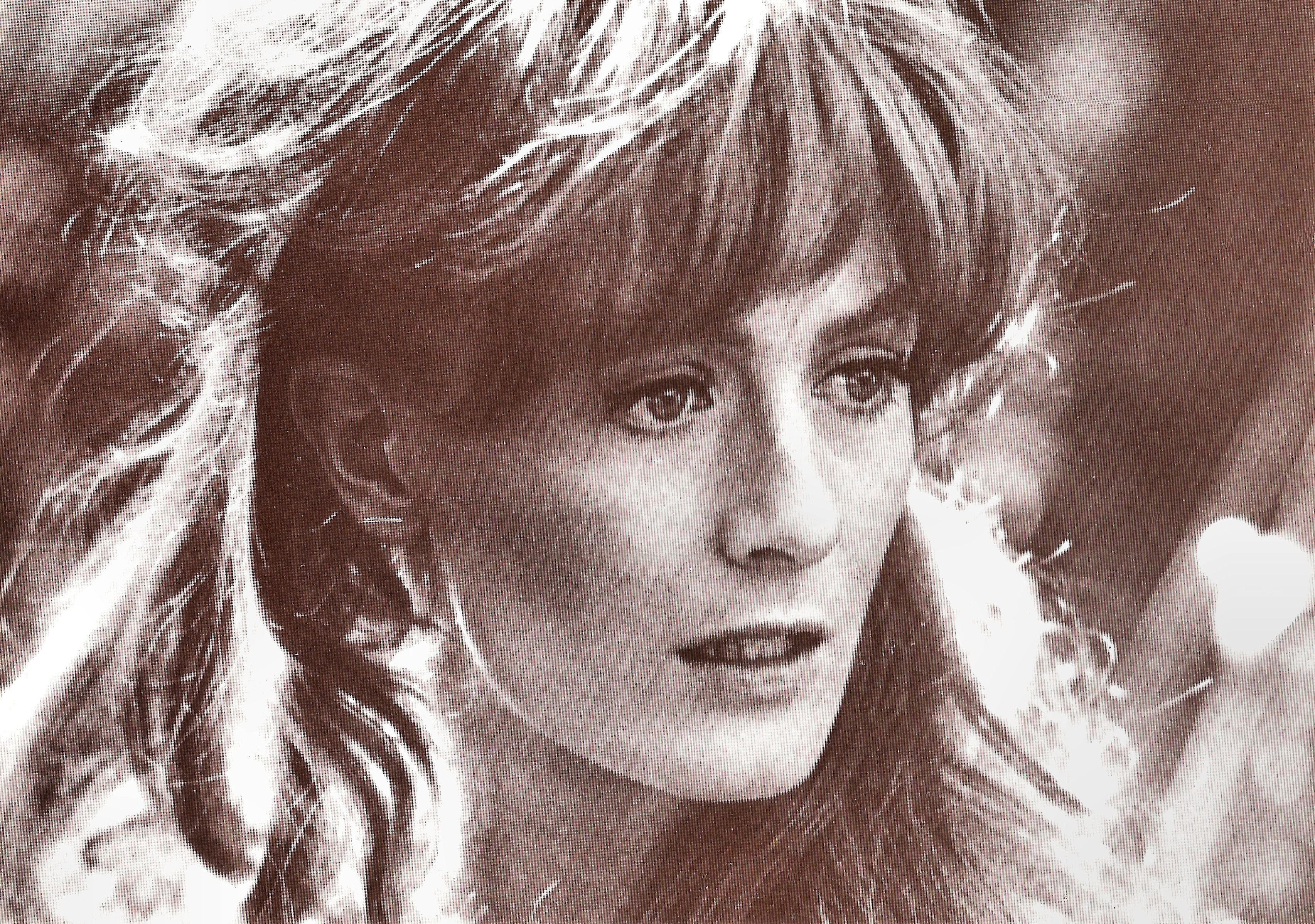This black and white image appears to be a screenshot from an older TV show or movie. It features a woman viewed from the neck up, sporting a 70s-style hairdo with long, wavy hair that extends a bit past her shoulders and straight bangs. Her dark, slightly curly hair catches the sunlight, which creates a glare and beams of light, especially illuminating the left side of her face and neck. The woman exudes a concerned or intense expression, with slightly open lips showing part of her top and bottom teeth. Her head is tilted, and her serious eyes gaze to the right. The image also highlights her pronounced right cheekbone and dark eyebrows. There is a blurry background, and no jewelry is visible, focusing the viewer's attention entirely on her contemplative face and hairstyle.